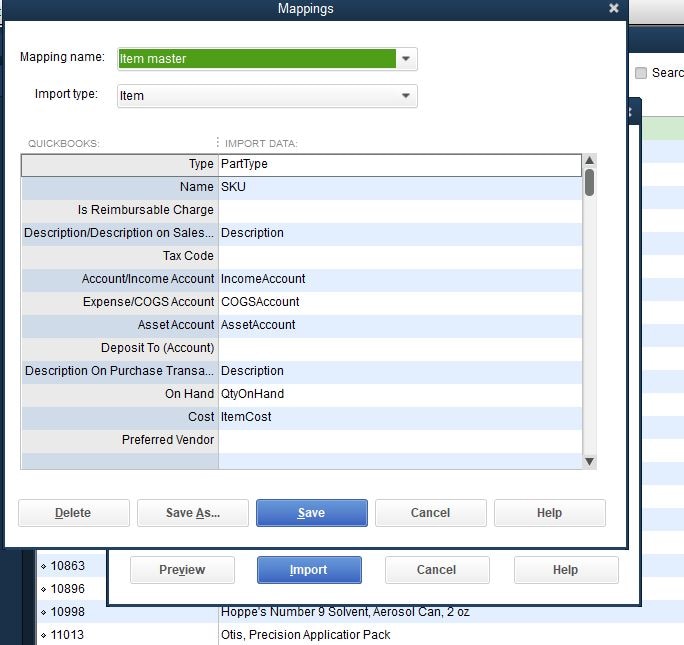The image depicts a detailed mapping screen interface designed for managing item imports into QuickBooks. At the top of the screen, a blue horizontal rectangle bar prominently displays the title "Mappings." Directly beneath, the interface categorizes entries with several dropdown boxes.

The first dropdown, labeled "Mapping Name," features a green box with white lettering that reads "Item Master." Below, another dropdown box is labeled "Import Type," displaying "Item" within a white box with black lettering. Two section headings are visible next: "QuickBooks" positioned to the left and "Import Data" on the right.

A detailed grid section follows, beginning with two main columns, “Type” and “Part Type.” Under "Type," entries include:
- Name
- SKU 
- Is Reimbursable 
- Charge 
- Each 

Alternating blue and white backgrounds enhance visibility across rows. Additional details are placed under "Part Type":
- Tax
- Description / Description on Sales
- Description as in Part Type
- Tax Code
- Account
- Income Account
- Part Type
- Income Account
- Expense
- COGS Account
- Part Type
- COGS Account
- Type
- Asset Account
- Part Type
- Asset Account
- Type Deposit to Account
- Description on Purchase Transaction
- Part Type Description
- Type On Hand
- Part Type Quantity on Hand
- Type Cost
- Part Type Item Cost
- Type Preferred Vendor

Further interface controls appear at the bottom, showcasing five buttons with different functions:
- Delete (white background, black lettering)
- Save As (white background, black lettering)
- Save (blue background, white lettering)
- Cancel (white background, black lettering)
- Help (white background, black lettering)

Below this set, another segment includes options for:
- Preview (white background, black lettering)
- Import (blue background, white lettering)
- Cancel (white background, black lettering)
- Help (white background, black lettering)

The bottom section features a list of item identifiers and names; for example:
- 10863
- 10896
- 10998
- 11013

To the right of these numbers, item descriptions include:
- HOPPES No. 9 Sullivan Aerosol Can, 2 ounces
- Otis Precision Applicator Pack

This comprehensive design aids users in efficiently configuring items for import into QuickBooks, ensuring detailed categorization and seamless data integration.